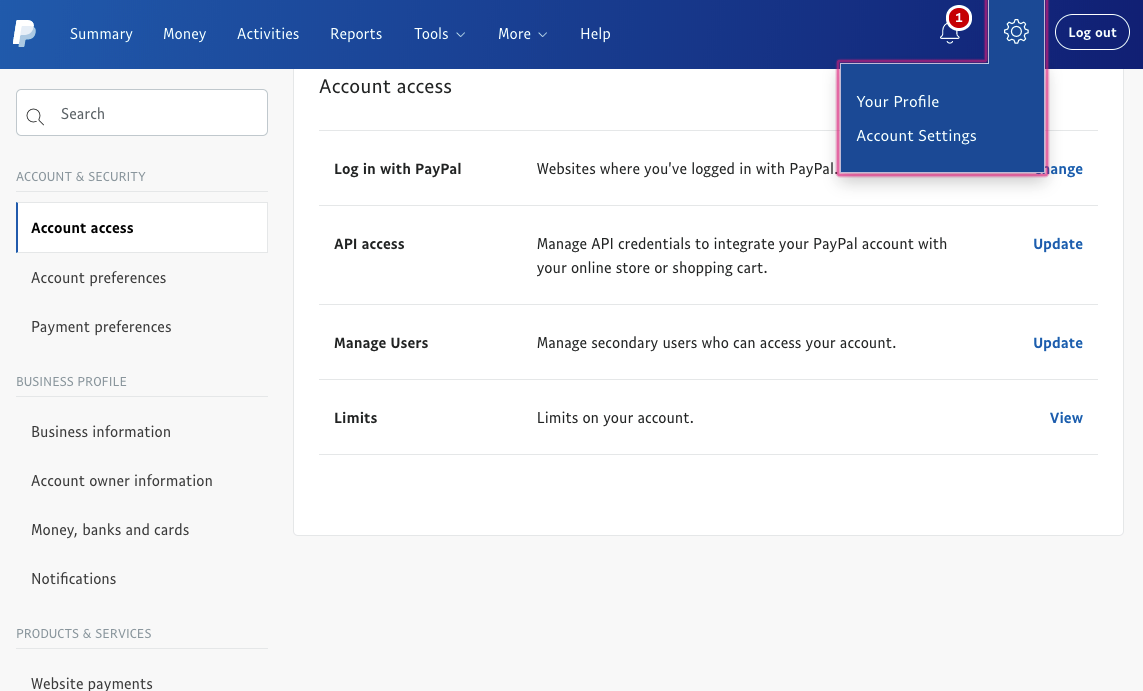In this detailed screenshot from a PayPal account, the familiar PayPal logo is prominent in the upper left-hand corner, accompanied by a variety of navigation tabs labeled Summary, Money, Activities, Reports, Tools, More, and Help. On the upper right side of the screen, there is a notification bell displaying the number "1," indicating a new notification. Adjacent to this is a settings button, which is notably highlighted with a red outline and reads "Profile and Account Settings." Nearby is the logout button for easy and immediate account exit.

The central content of the screenshot is divided into various sections. The first section, titled "Account Access," provides options for "Login with PayPal" and includes a button to manage websites where the user has logged in with PayPal. The second section, "API Access," offers information about managing API credentials to facilitate integration of the PayPal account with an online store’s shopping cart, accompanied by an Update button.

Next, the "Manage Users" section allows for the management of secondary users who can access the PayPal account, with the available action being an Update button. The final section, "Limits," displays any account limits, offering a View button for more detailed information. Each section is meticulously structured to offer clear, actionable steps for various account management tasks.